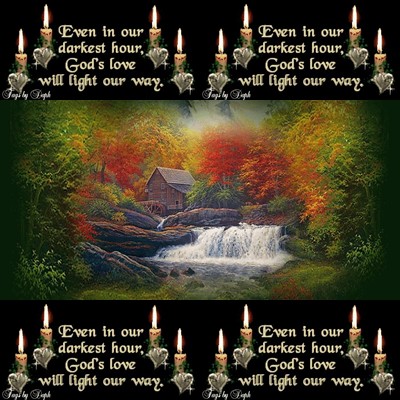This image resembles an inspirational meme or a postcard with a tranquil, autumn-themed painting reminiscent of Thomas Kinkade's works. Dominating the scene is a picturesque wooden cabin or farmhouse, nestled amid vibrant autumn foliage that transitions from green at the edges to rich reds, oranges, and yellows towards the center. A small, serene waterfall flows in the foreground, adding to the peaceful ambiance. The image is framed by letterbox-style black bars at the top and the bottom. Within these bars, the message, "Even in our darkest hour, God's love will light our way," is elegantly repeated four times in a flowy, ornate white font. Each iteration of the text is accompanied by an image of a glowing candle, placed at the corners of the black bars, enhancing the comforting and uplifting message.